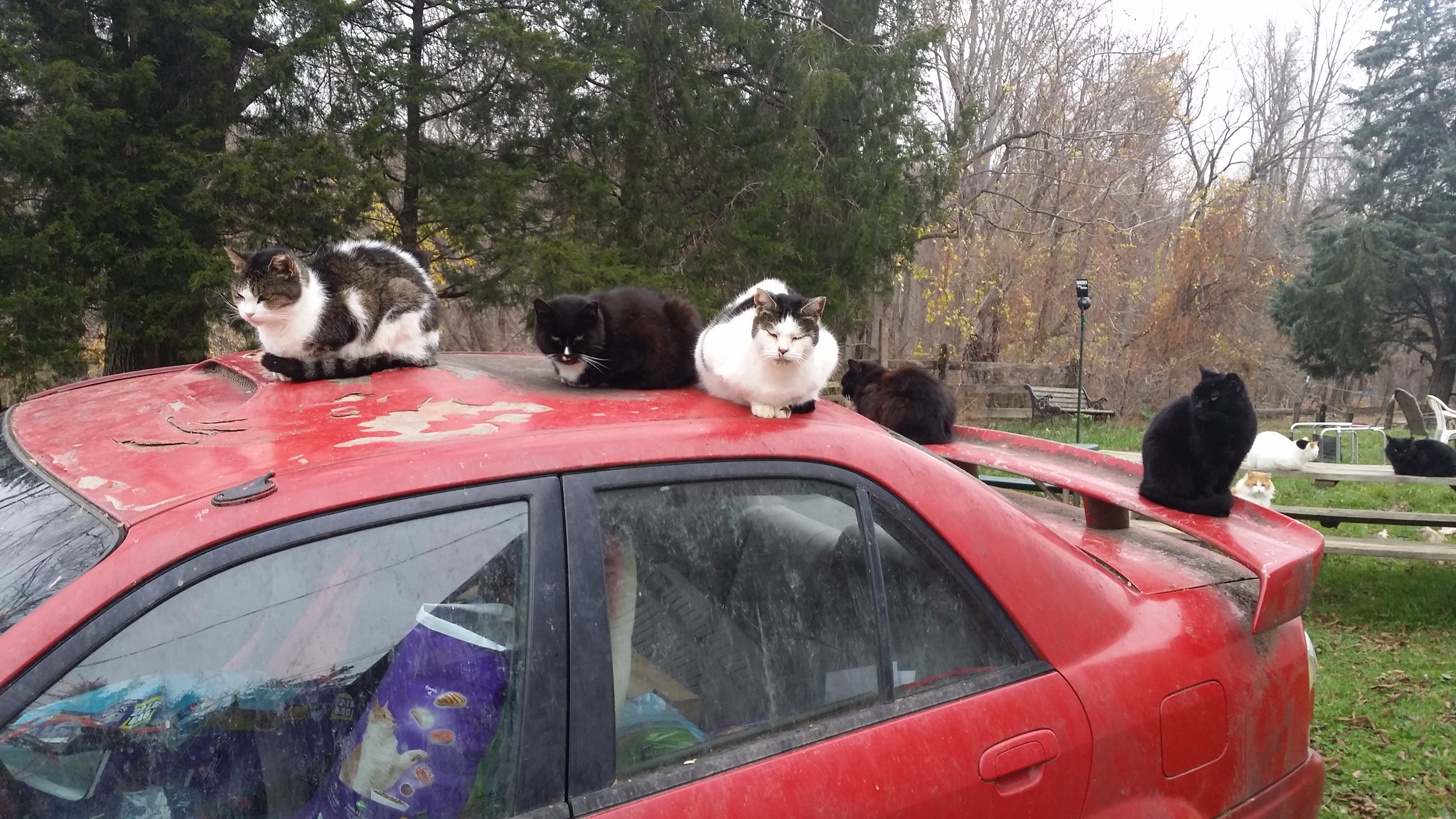This color photograph, taken outdoors during a fall day in a city park, showcases a slightly run-down red car with a spoiler on the back. The car is parked on a grassy area amidst trees with leaves turning golden. On the hood of the car are three cats: a white and gray one, a black and white tuxedo cat with a distinctive white spot on its nose, and another white and gray feline. Two more cats, both primarily black, are lounging on the spoiler. The interior of the car is cluttered, notably with a large bag of cat food visible on the driver's seat, indicating it might be a gathering spot for these felines. In the background, park benches host additional cats, including a white and caramel one on the seat, a mostly white cat with some colored markings on its head, and another black cat on top of the bench. Further details show a few patio chairs and more cats on a distant fence, emphasizing this area as a popular haven or colony for cats.